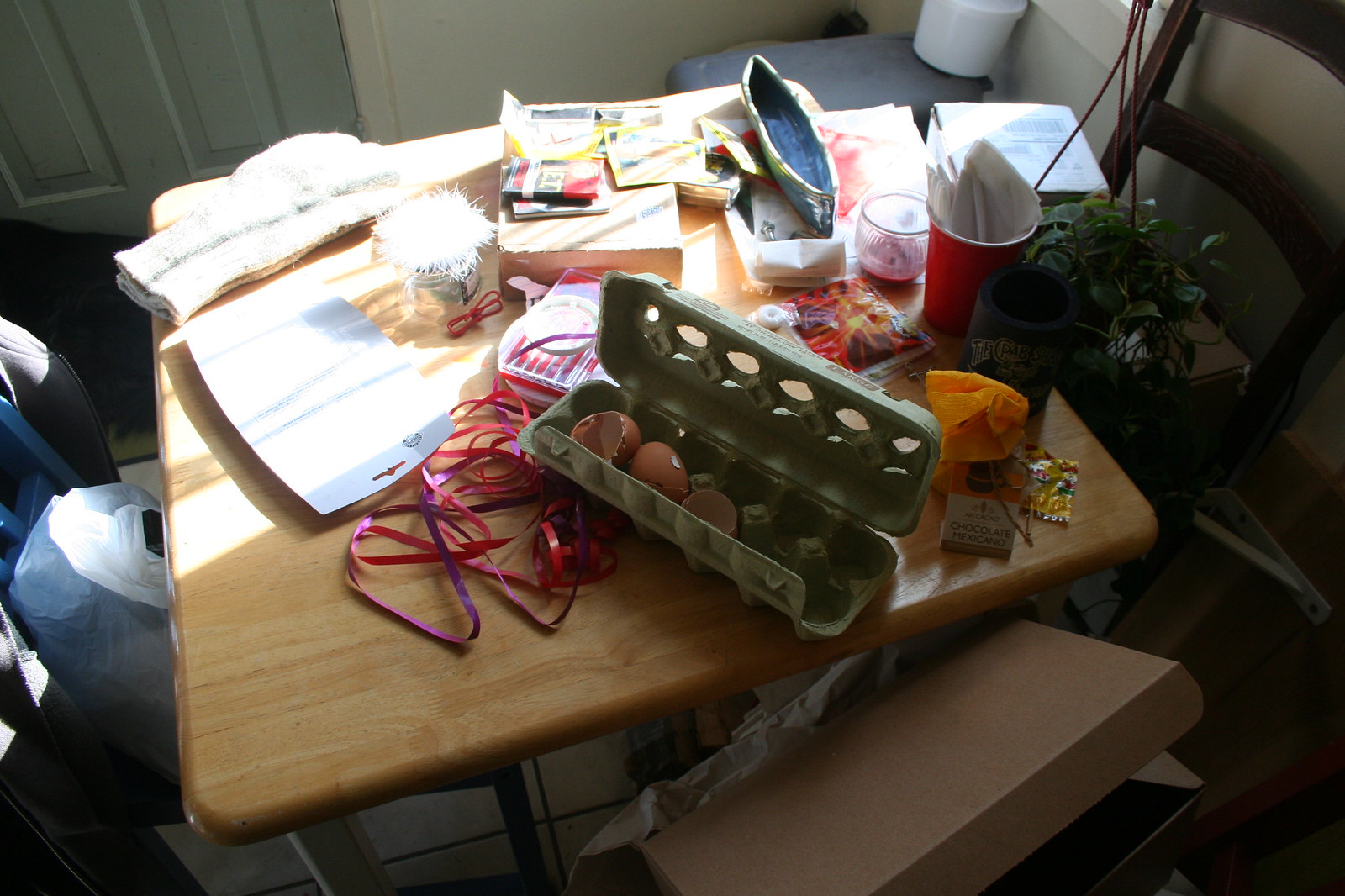This image depicts a highly cluttered room with a central focus on a table. The table originates from the bottom-left corner of the frame, extending at an angle to the right before sharply bending back towards the left amid piles of clutter, ultimately reaching near the top center and then veering left and descending back down. 

The upper part of the scene reveals a slice of a green door at the top-right, adjacent to a white wall. In the middle field of view, there is a faint sight of a gray object behind a white bucket in the background corner. Underneath the table, portions of the white-tiled floor are visible. Slightly to the right of the table stands a blue chair partly visible, with a white bag perched upon it.

Light floods in from a window on the right side, casting illumination on the top-left corner of the table. The table itself is draped in a blue tablecloth. Atop this, a white cutting board is placed. To the right of the cutting board, there is an indistinct, fuzzy object. A box topped with papers lies next to it, followed by an open purse with a silver side pointing downwards, resting on additional papers. Near the edge of these papers is a pink candle. Further down and to the right, a red Solo cup filled with papers and pens stands next to a black beer koozie.

Near the right edge of the table, a plant ascends from beneath beside the back of a brown chair. A little below and to the right of the beer koozie, an orange bag containing chocolate lies. Just left of this bag, a carton turned sideways displays three broken eggs, with the rest of the compartments empty. Bright yellow and red streamers are partly visible beneath the carton. At the bottom center extending upwards to the right, a box wedges into view.

This room captures a chaotic scene, filled with an eclectic mix of personal items scattered across the table and surrounding area.